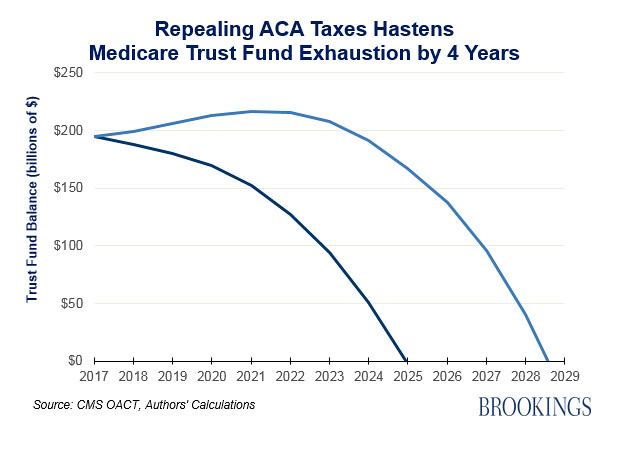The image is an infographic with a landscape orientation, depicting a detailed line graph titled "Repealing ACA Taxes Hastens Medicare Trust Fund Exhaustion by Four Years" in bold blue letters at the top. The y-axis, labeled "Trust Fund Balance (Billions of Dollars)," ranges from 0 to 250 in increments of 50. The x-axis spans the years 2017 to 2029. The graph includes two blue lines: a darker blue line declining steeply to zero by the year 2025, and a lighter blue line extending to mid-2028 before reaching zero. The bottom right corner of the graph features the word "Brookings," and the bottom left corner notes the source as "CMS OACT, Author's calculations." The lines and text collectively illustrate how repealing ACA taxes accelerates the depletion of the Medicare trust fund.